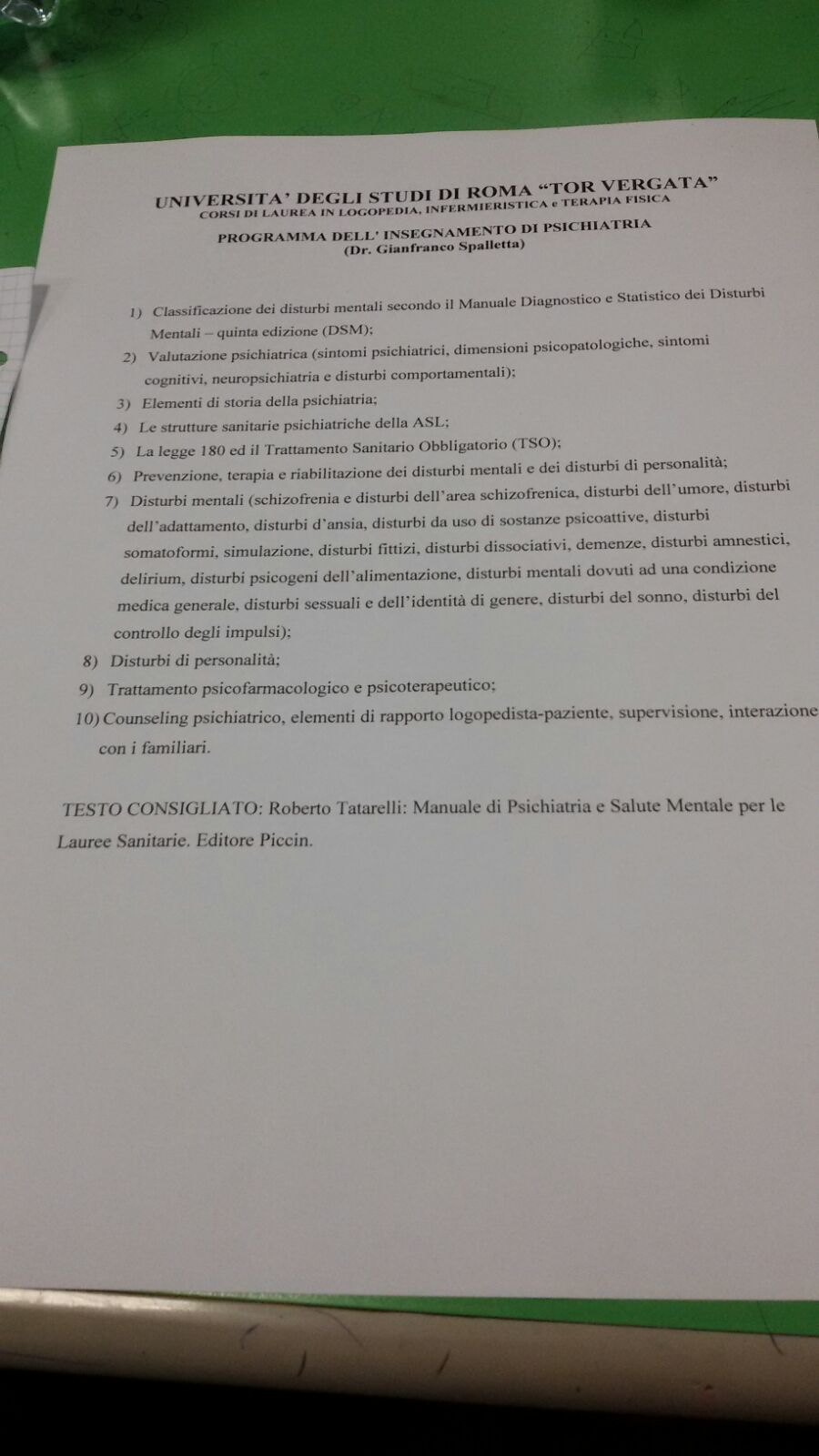This photograph depicts a piece of white paper with printed text, resting on a shiny green glass tabletop that has a gray, rounded plastic edge. The top section of the paper features a bold, all-caps title that reads "UNIVERSITA DEGLI STUDI DI ROMA TOR VERGATA," indicating that the document is likely written in Italian. Below the prominent title, a series of lines in much smaller fonts are printed, though they are illegible in the image. The paper continues with a number of vertically aligned, numbered bullet points—approximately 15 to 20—that are also too small to be read clearly. Another piece of paper partially overlaps the bottom left corner of the main paper, casting a slight shadow. At the bottom of the document, in uppercase letters, it reads "TESTO CONCILIATO," followed by more unreadable text in lowercase letters. The overall setup gives the impression of a formal document, possibly an important schedule or set of instructions, arranged on a distinctive green tabletop with a reflective surface.